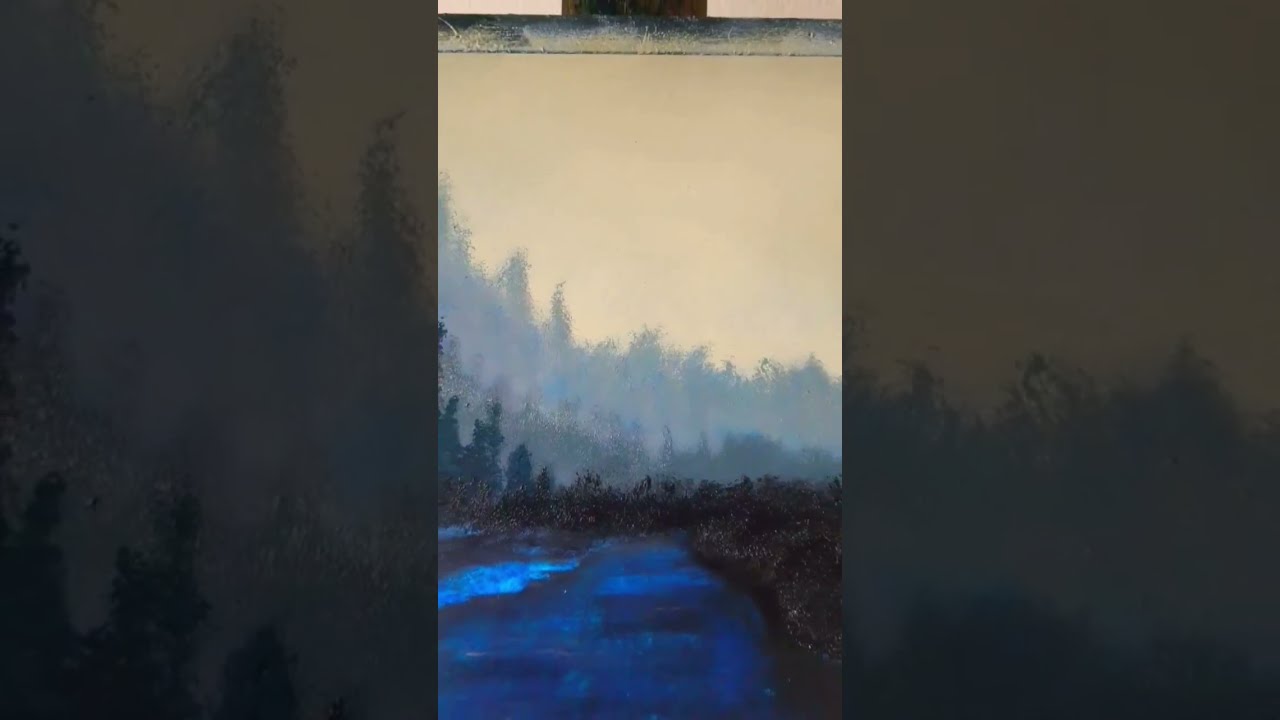The artwork is an oil painting on canvas, depicting a serene nature scene. The foreground features a deep, dark blue body of water, possibly a lake or creek, with hints of white caps or gentle waves adding texture. Surrounding the water is a green shoreline that wraps around to the left, punctuated by tall, brown weeds on its bank. Layers of forest, with poofy green pine trees, create a sense of depth as they ascend a sloping mountainside that descends toward the right. The background reveals a hazy, muted orange and yellow off-white sky, suggesting an early morning or late evening scene. At the very top center of the painting, the canvas is mounted on an easel, visible as a horizontal pole with a small rectangular square on top, reminding viewers of its artistic creation.